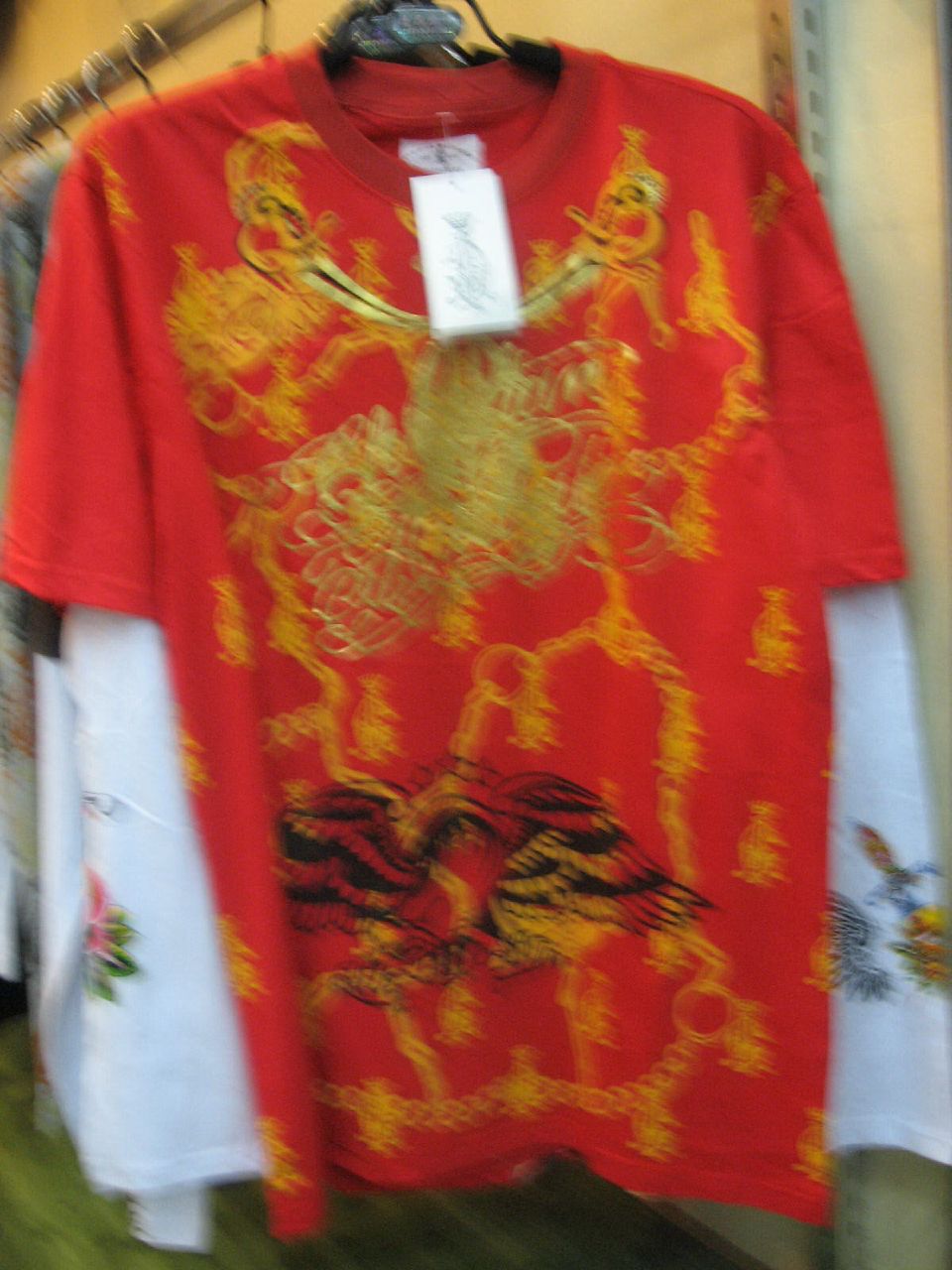This somewhat blurry photograph captures a rack of clothing with items hanging on hangers. At the forefront is a striking ensemble featuring a bright red, short-sleeved, crewneck t-shirt layered over what appears to be a long-sleeved white shirt, or possibly just the white sleeves are visible. The red t-shirt is adorned with an intricate gold and yellow design on its front, which incorporates elaborate patterns and shiny gold letters, although the text is indistinguishable. The bottom part of the shirt displays a stylish black bird motif with its wings spread wide.

Extending from beneath the t-shirt are the long, wide cuffs of the white sleeves, embellished with what seems to be an embroidered floral design. A white price tag dangles conspicuously from the t-shirt's collar. In the background, the clothing rack holds several more garments, all arranged against a cream-toned, stone-like wall. The combination of vivid colors, intricate details, and layered garments creates a captivating focal point in the image.